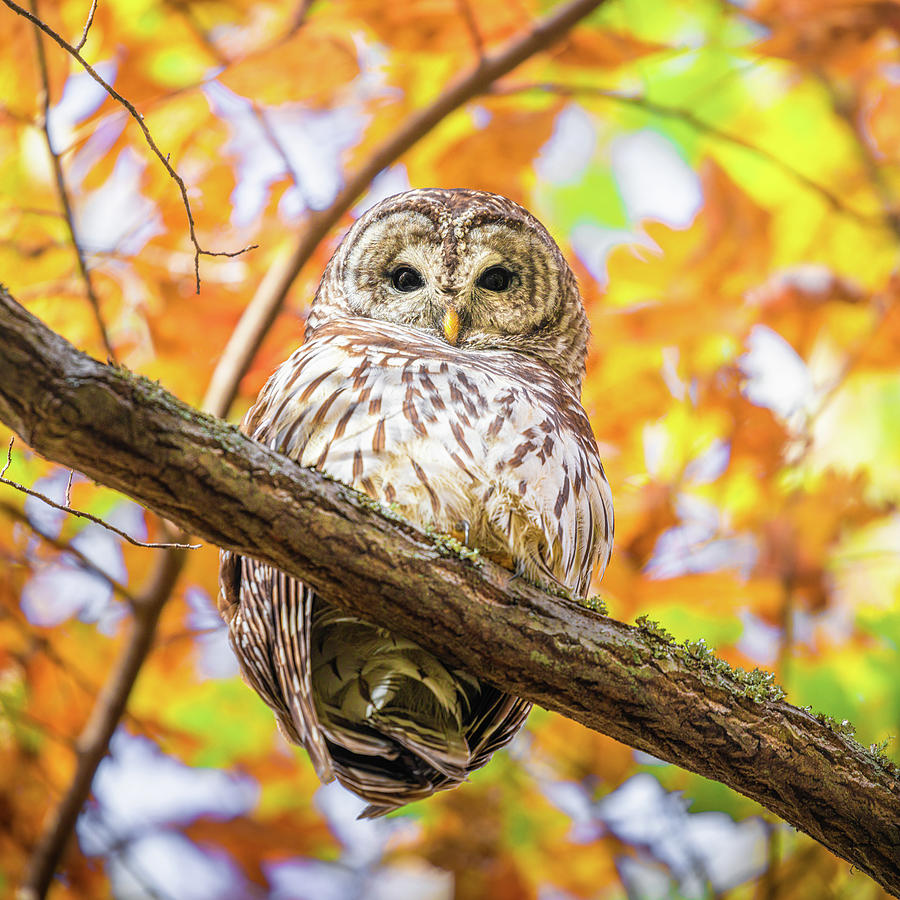The photograph captures a beautifully perched owl on a gray-brown tree branch adorned with light gray-green lichen. The owl, a mesmerizing mix of white, gray, and brown speckled feathers, sits in the center of the image, gazing directly at the viewer with its dark, almost-black eyes and small yellow beak. The camera angle looks up at the owl, revealing its underside, tail, belly, and curious face. The tree branch extends horizontally at an upward angle towards the left and downward towards the right. The blurred background, suggestive of digital art, features a vibrant autumn palette of golden and orange leaves, accented with light green and patches of light blue sky. The overall image is bright and evokes a peaceful, serene atmosphere, capturing the owl's tranquil yet inquisitive demeanor amidst the autumn foliage.